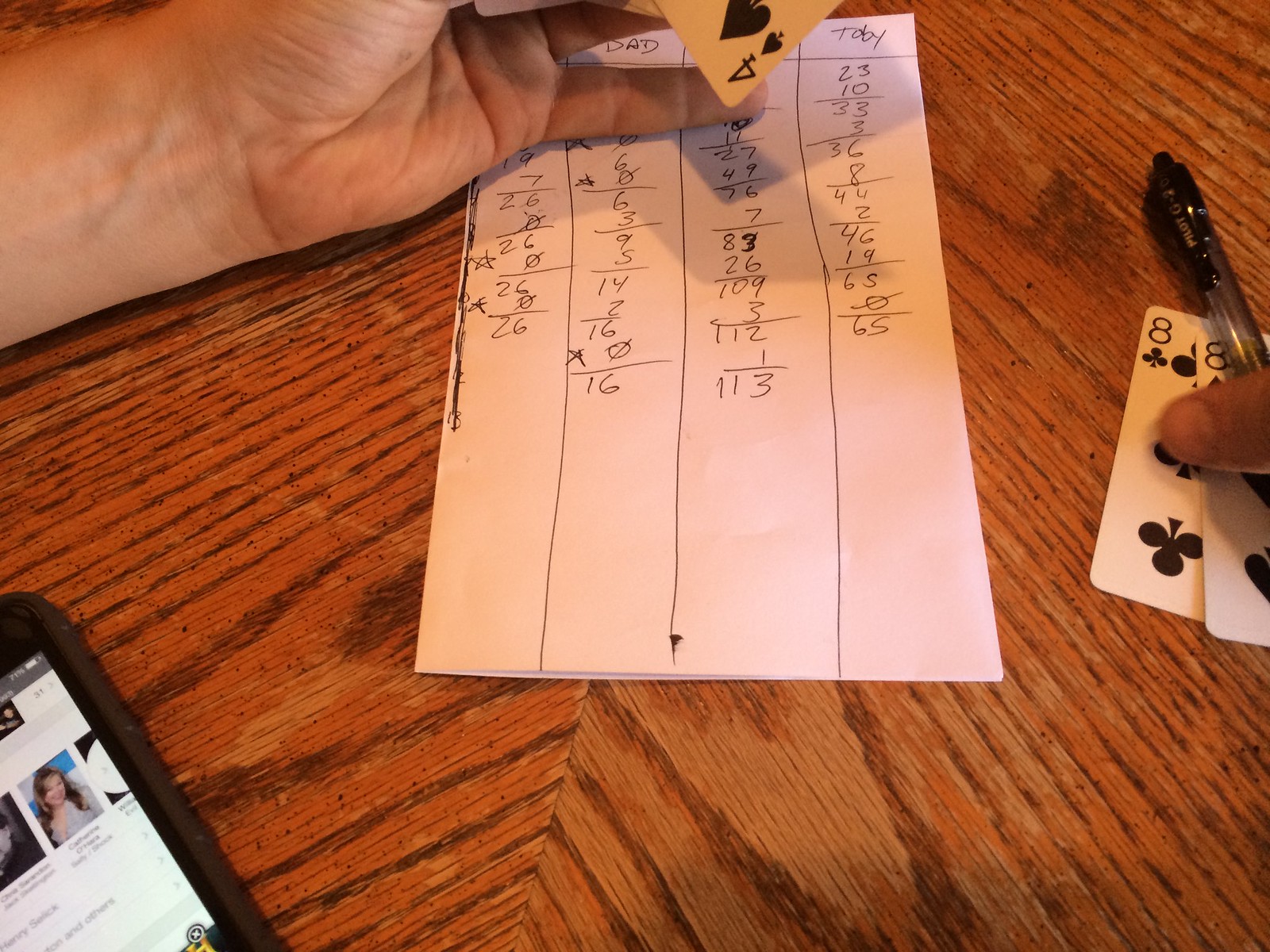This image captures an intimate scene of a well-worn, brown wooden table, bearing the marks of extensive use, presumably as a heart of social and intellectual activity. Situated atop this table are the hands of a card player, seen from their own perspective, indicative of a game in progress, possibly Bridge. The player's left hand is prominently visible, clutching a set of cards, revealing just a glimpse of the four of spades. Meanwhile, the right hand is partially obscured, with either a finger or thumb resting on two face-up eights laid on the table. These cards are intersected by a pen, subtly hinting at the analytical nature of the game.

In the center of the image lies a narrow sheet of paper oriented vertically, serving as a scorecard. This scorecard is divided into four columns, listing the participants. The name "Toby" is discernible in the far-right column, "Dad" occupies the second-from-left, while the remaining two columns are not entirely visible. The lower left-hand corner of the image partially includes a smartphone, its display illuminated and facing upwards, suggesting its use either as a timer, scorekeeper, or perhaps a means to refer to rules or strategies.

This meticulously detailed portrayal encapsulates the ongoing interaction, evoking the strategic and social essence of the moment, with all elements pointing towards a game of Bridge being played.